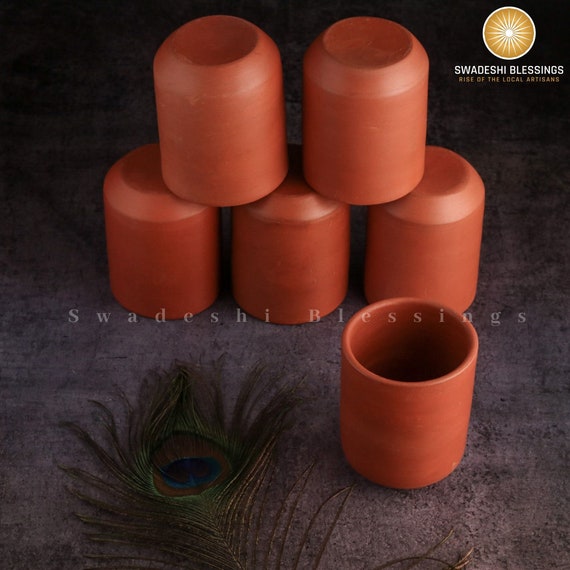The image shows a set of artisan clay cups with a warm reddish-brown terracotta color, reminiscent of traditional flower pots. In the composition, five cups are turned upside down in the background—three on the bottom row and two more stacked on top of them—while a single cup sits upright in the foreground towards the bottom right. The setting features a dark brown or charcoal gray table that complements the earthy tones of the cups. 

In addition to the ceramic pieces, a dark peacock feather is positioned near the bottom center of the image, subtly blending into the background. The feather displays various shades of green, with a striking central eye pattern featuring a blue circle encased in a brown splotch. 

Text elements include the phrases "Swadish Blessings" and "Rise of the Local Artisan," displayed centrally in gray and also located in the upper right corner inside a yellow sun-like circle. The rich color palette of the image includes earthy reds, greens, blues, and warm neutrals, all contributing to an artisan and handcrafted aesthetic.